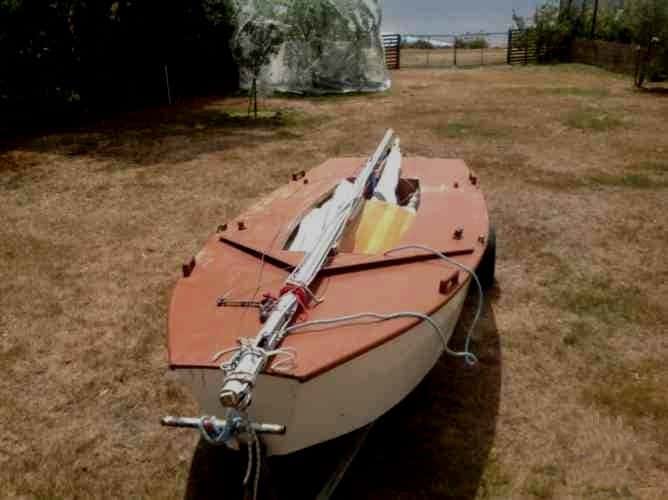The image displays a small sailboat situated on dry, parched grass that is predominantly brown with sparse green patches, suggesting the yard has seen better days. The sailboat, which features a red top and a white lower hull, is clearly not in use, as its mast is folded down and secured flat along its length with ropes. The open area on the boat indicates that it is prepared for storage rather than sailing. The backdrop includes several trees and a fence, beyond which a body of water is just barely visible, hinting that the location might be near a lake. However, the immediate surroundings, which contain pastoral elements like the fence typical of a farm or backyard, and a dark, looming structure on the left, emphasize the landlocked setting. The quality of the photograph is somewhat blurry and grainy, adding to the rustic feel of the scene.